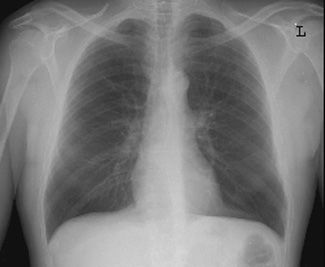This image is an x-ray of a human chest, featuring a small capital letter "L" in the upper right corner to indicate orientation. The background is black, highlighting the white depiction of the bone structures, including the clavicle, ribs, spine, shoulders, upper arm bones, and parts of the upper leg bones. The chest cavity reveals clear lungs, though there is a slightly transparent, pale area in the middle center of the lungs that could signify an abnormality. The spine is faintly visible running from the top to the bottom of the image. The image is slightly blurry but distinctly shows the various bones and organs within the torso.